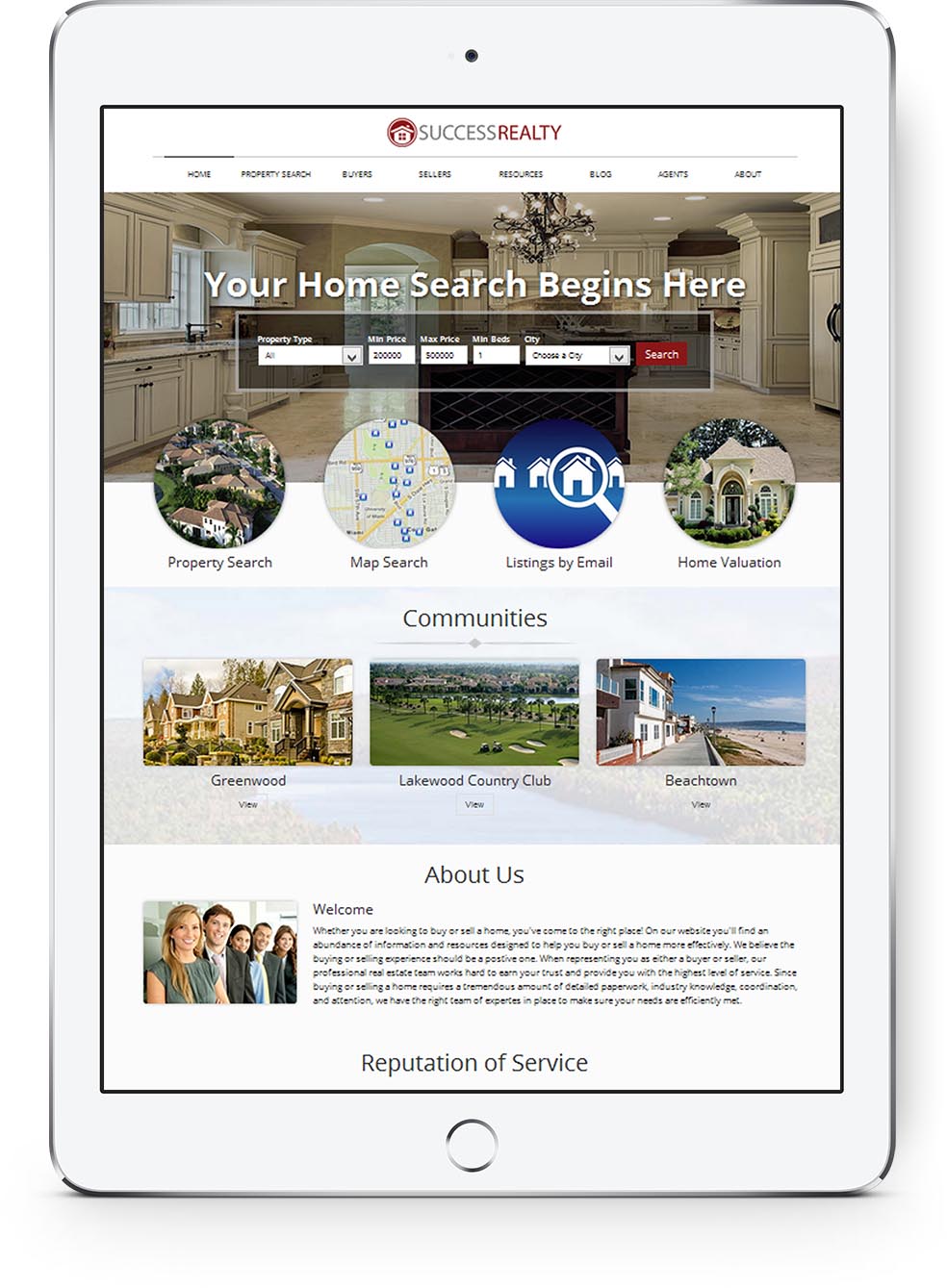The image depicts a vertically oriented, rectangular device resembling an iPad, characterized by a thin silver border that encloses the frame. This border encompasses a white backdrop that extends uniformly around the screen. The upper middle section of the device features a black circle, and the lower middle section houses another circle distinguished by a black ring with a white center, identified as the home button.

Centered within the iPad's display is a red emblem with a white house symbol inside, accompanied by the text "Success Realty." Below this emblem lies a horizontal navigation menu with labeled options: Home, Property Search, Buyers, Sellers, Resources, Blog, Agents, and About.

Further down, the screen showcases a large image of a modern kitchen. The kitchen is notable for its white cabinetry and tiled surfaces and includes a central island, which may function as a wine holder. Superimposed on this kitchen image are the words "Your Home Search Begins Here." Directly beneath this text is a search box designed for entering home-related criteria such as property type and price, accompanied by a prominent red "Search" button.